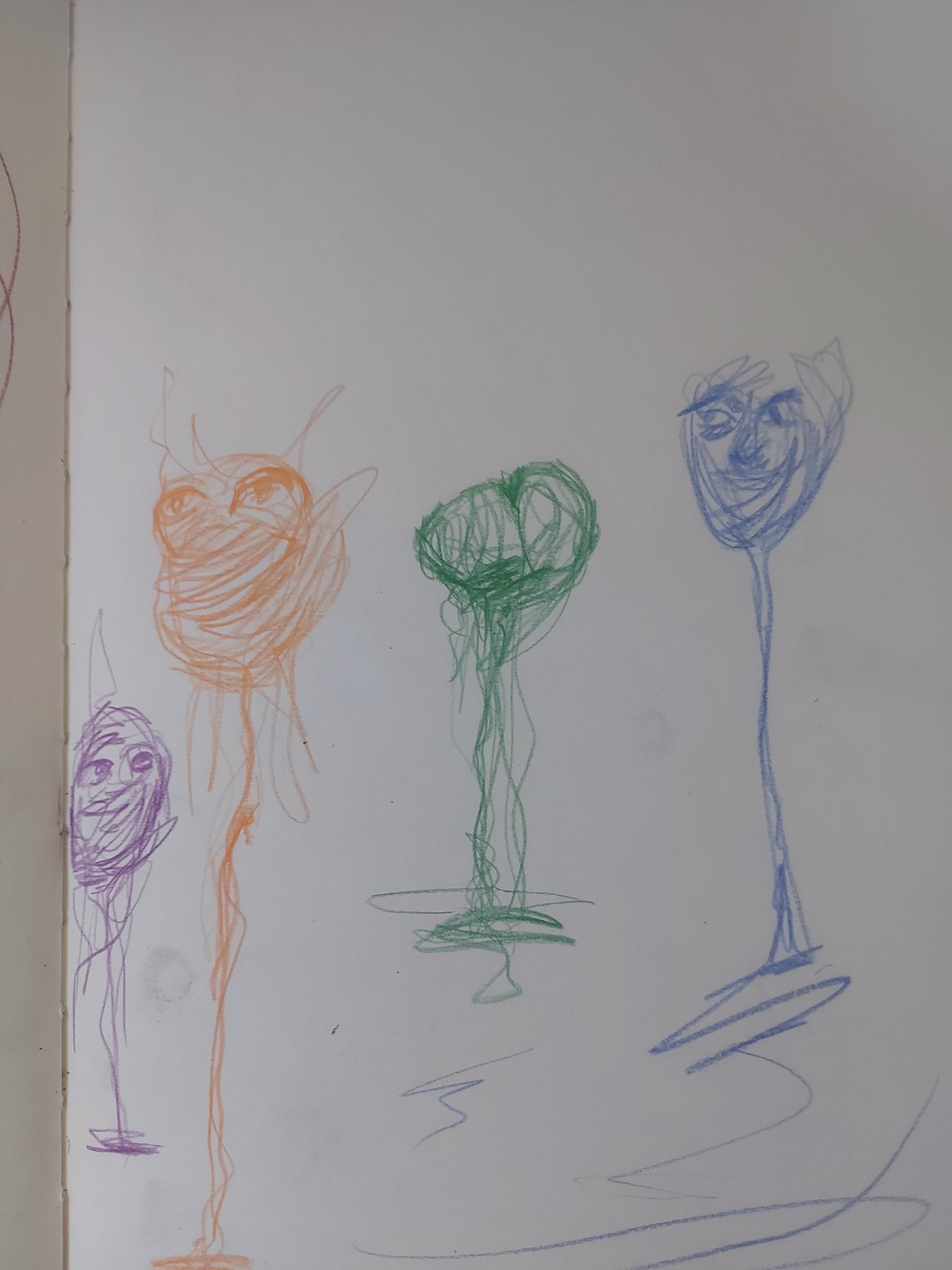The image depicts a white sheet of drawing paper adorned with four colorful character sketches. Each character features a head-like form situated atop a straight, stem-like line. Starting from the left, the first drawing is in purple, with big eyes, a discernible nose, a straight-line mouth, and squiggly hair, although the body is merely a straight line with a small squiggle at the bottom. The next character, in orange, is significantly taller, also having a straight-line body; it's difficult to make out facial features here. Continuing right, the third character, in green, has a short stature with a nearly heart-shaped form and no recognizable face. The final character, in blue, is taller than the green one but shorter than the orange, showing clear facial features including eyes, eyebrows, and a smiling mouth. Each character's head sits atop what resembles the stem of a wine glass, contributing to a whimsical and abstract representation.